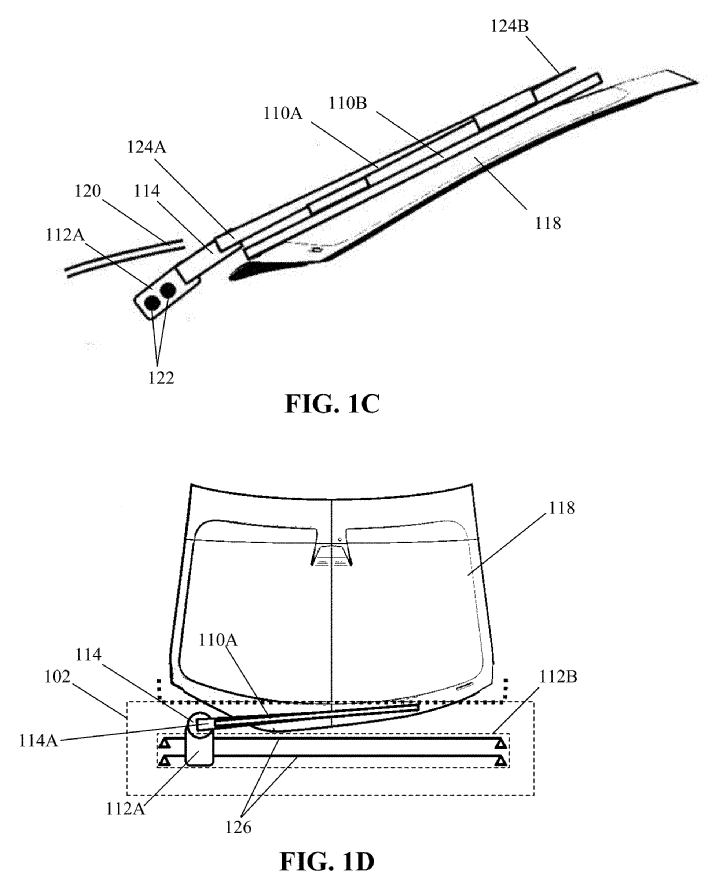The image features two black-and-white hand-drawn figures labeled 1C and 1D. Figure 1C presents a side profile of a thin, elongated object that closely resembles a windshield wiper, with two dark spots at its base suggesting connection points. Adjacent to this object is a blade-like structure. Figure 1D emphasizes the object's placement, depicting it in what appears to be an unsymmetrical car hood area, potentially indicating where this oblong item might fit. Both figures are densely annotated with corresponding numbers in the 100s, identifying various sections of the diagram. Despite these details, the exact nature of the illustrated item remains ambiguous as no explanatory text accompanies the diagram, leaving the identity and context of the object open to interpretation.